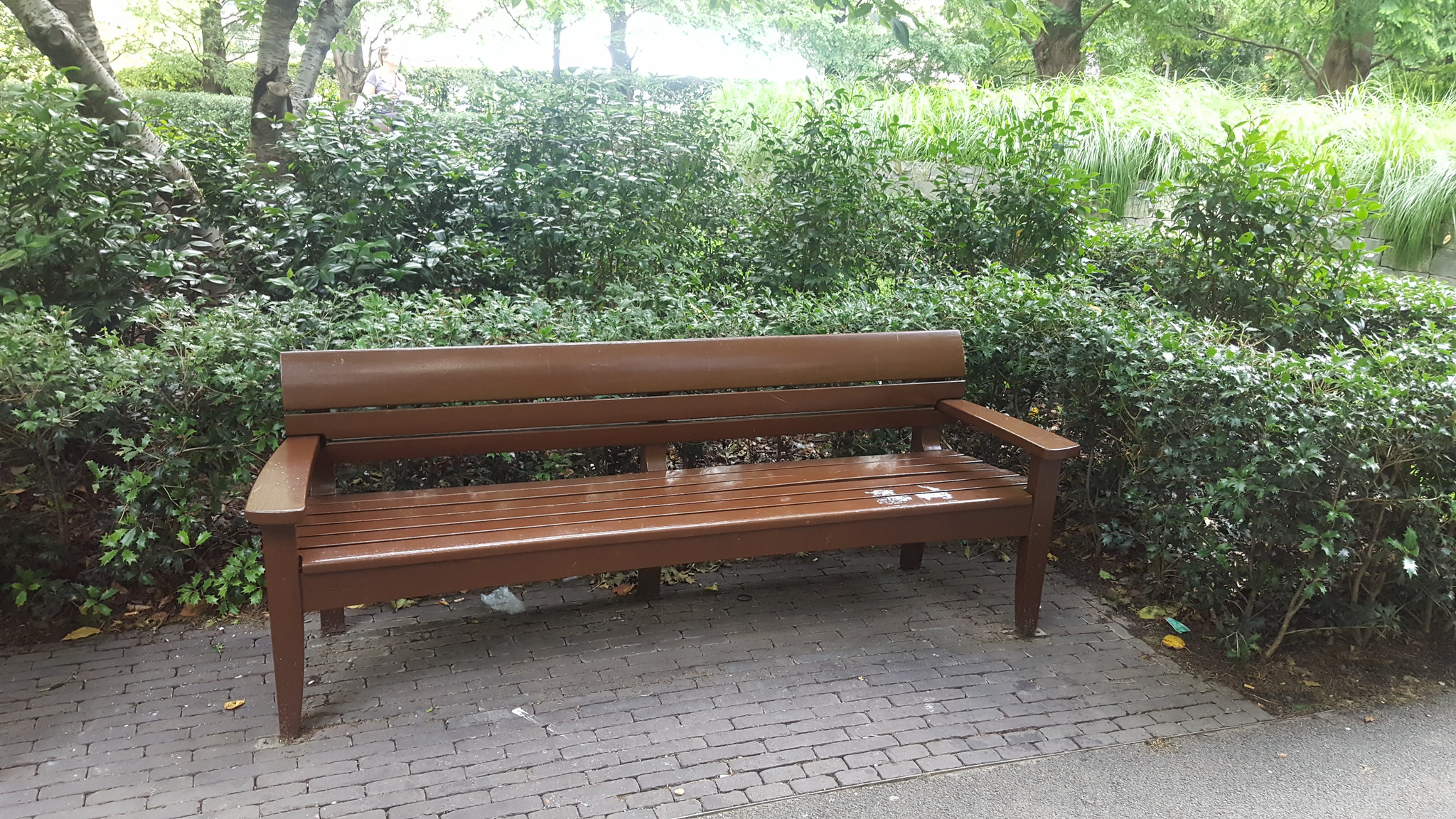The photograph depicts an outdoor scene featuring a polished, brown wooden bench with slats on both the seat and backrest. The bench, which could comfortably seat three to four people, is situated on a base of slightly weathered, red-gray brick pavers. Surrounding the bench is a semi-wild yet well-kept array of lush green hedges and various foliage, including some higher plants and the trunks and branches of trees in the background. The area is bright, with sunlight filtering through the leaves, contributing to a vibrant and lively atmosphere. To the right and lower right of the brick area, there is a gray asphalt or concrete walkway. Scattered leaves and a possible piece of discarded paper lie on the ground around the bench, adding to the natural feel of the scene. Overall, the image conveys a serene spot in a park or garden where one could sit and enjoy the beauty of the outdoors.